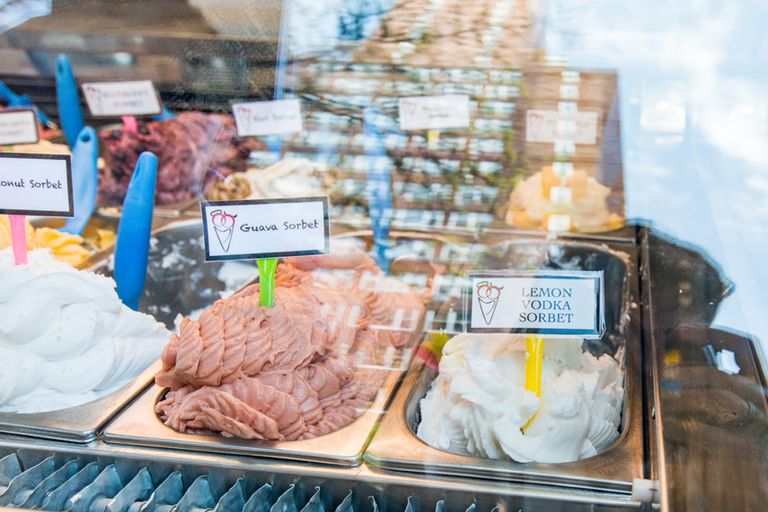The photo depicts a display case in an ice cream or sorbet shop, showcasing a variety of sorbets housed in metal containers behind protective glass. The display case holds about a dozen sorbets in two rows, though the reflections on the glass obscure the view of those in the back. The three visible flavors include Coconut Sorbet, which is nearly pure white, Guava Sorbet, a natural pink hue, and Lemon Vodka Sorbet, also white. Each sorbet has a little label with its name, barely readable due to light reflections. Blue handles or spoons are present in each sorbet, adding a touch of color to the otherwise understated palette. The reflections reveal someone holding a camera, capturing the flavor options in this inviting shop setting.